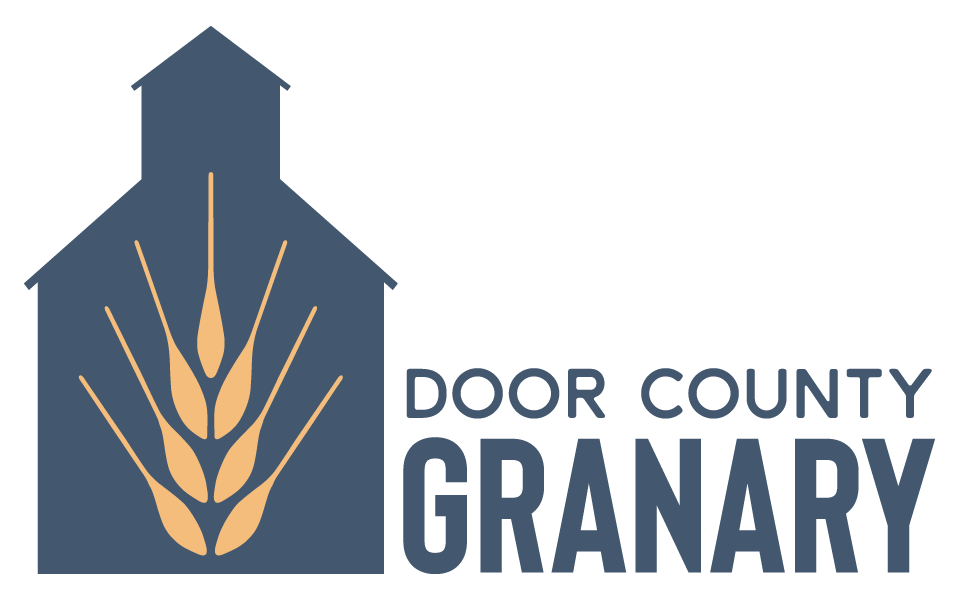This is an advertisement for Door County Granary, prominently featured with blue text. "DOOR COUNTY" is written at the top in all capital letters, followed by "GRANARY" in a larger font beneath it. On the left side, there's a blue silhouette of a distinct building resembling a barn. The structure starts with a rectangular base, then slopes inward toward another smaller rectangular section at the top, culminating in a pointed roof. Inside the silhouette, there are stylized depictions of grain stalks, resembling long spoons, with three on each side facing upwards and one in the center pointing downwards, all in the same light blue color as the text. The background is a solid white, making the blue tones and detailed design stand out.